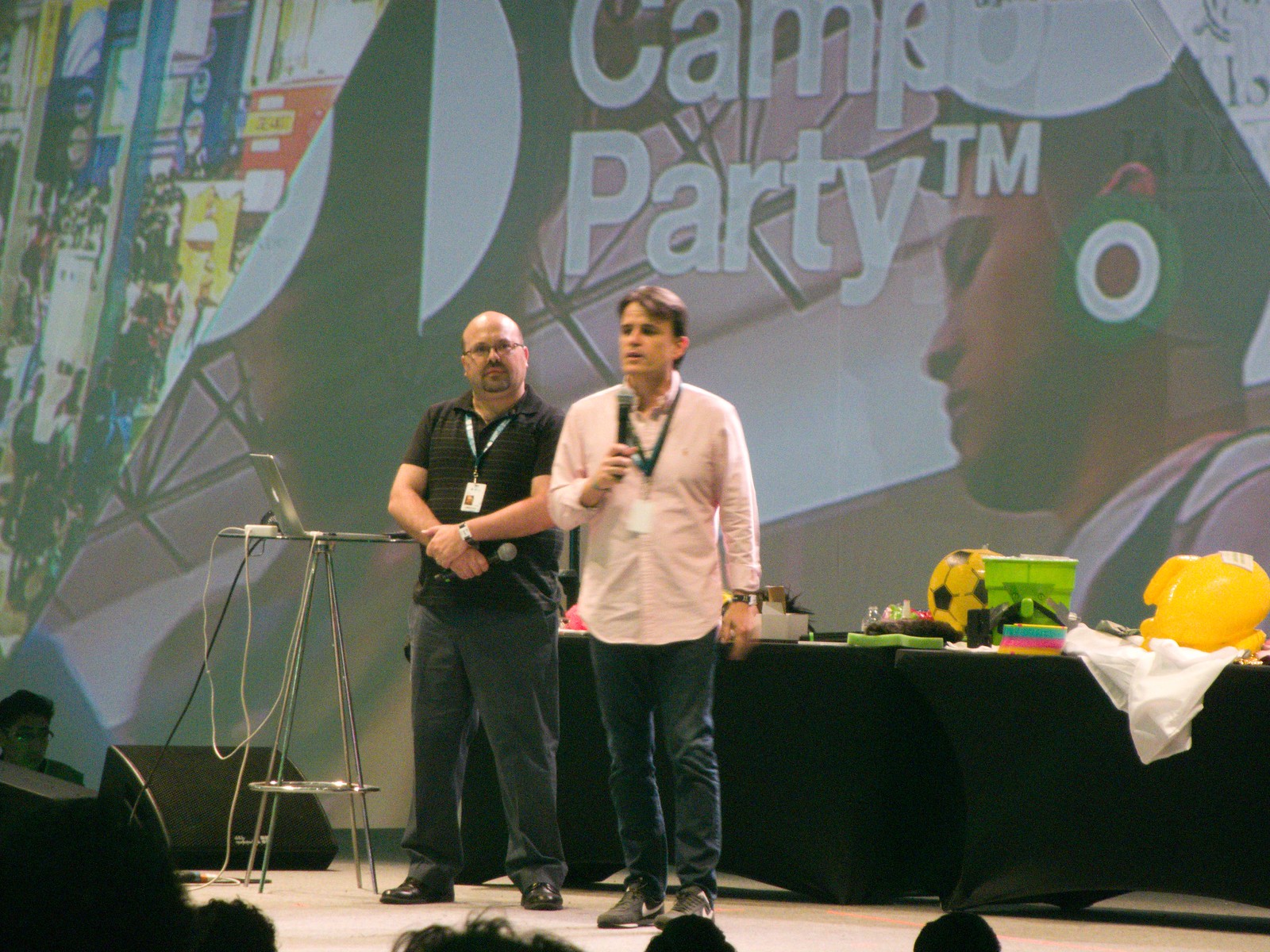Two men are standing on a stage, engaged in a demonstration or presentation. The man speaking into a microphone appears to be middle-aged and is dressed in a long-sleeved, untucked collared shirt—described as either pink or white—and blue jeans, complemented by Nike sneakers. He also wears a blue lanyard around his neck. Next to him stands a slightly heavy-set man with a bald head, wearing a dark polo shirt, a blue lanyard, baggy blue jeans, and dress shoes. He has his hands clasped in front of him and is looking attentively at the speaker. A sleek podium or table with an open Apple laptop is positioned near them. Behind them is a table draped in a black tablecloth, adorned with a selection of colorful items, including an inflatable yellow soccer ball, a beach bucket, an inflatable rocket ship, and other toys. On the wall behind them, a projection displays the text "Camp Party™."